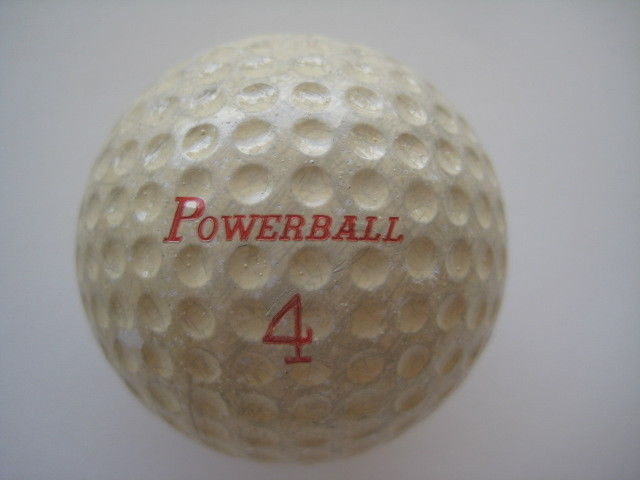This photograph is a close-up of a slightly off-white, dingy golf ball, prominently featuring small, circular indentations typical of a golf ball's surface. The ball is centered and fills most of the image. Across the middle of the ball, in uppercase red lettering, the word "Powerball" is written, followed by the number "4" just below it. The background is a smooth, gradient gray that transitions from medium gray at the edges to lighter gray towards the center, emphasizing the golf ball. The image has a dated, old-fashioned feel, suggesting it could have been taken years ago. Despite being zoomed in, the worn and used condition of the ball is evident, adding to the overall character of the photograph.